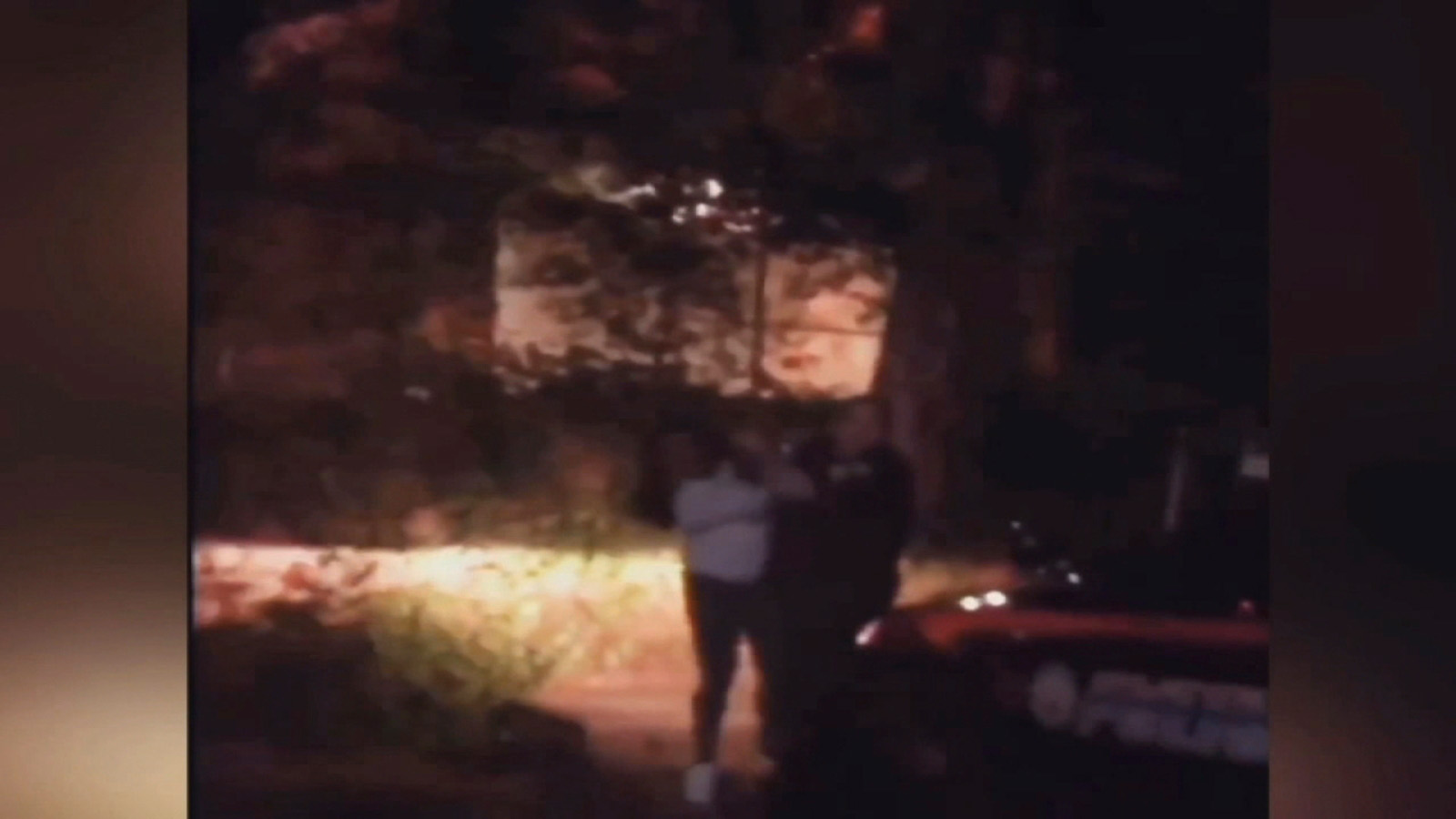This nighttime, outdoor photograph, seemingly captured from a dashcam or surveillance camera, is heavily blurred and grainy. The scene is dominated by a palette of dark browns and blacks, with a few distinguishable elements illuminated by scattered yellow lights. Central to the image are two figures standing near a reddish, shiny car. The car, which appears to be a police vehicle, has white writing partially visible, showing letters like "P" and "O."

Amidst the scene, tree branches and foliage are visible, their leaves rendered indistinct by the blur. There's a faint glow around a house with a large window seen behind the scene, partially concealed by the trees. The figures include a person in a white shirt with black pants and white shoes, seemingly engaged in a struggle or confrontation with two individuals in black uniforms, indicating a possible interaction with police officers. One officer is discernibly white, while the other details remain obscured by the photo’s poor quality.